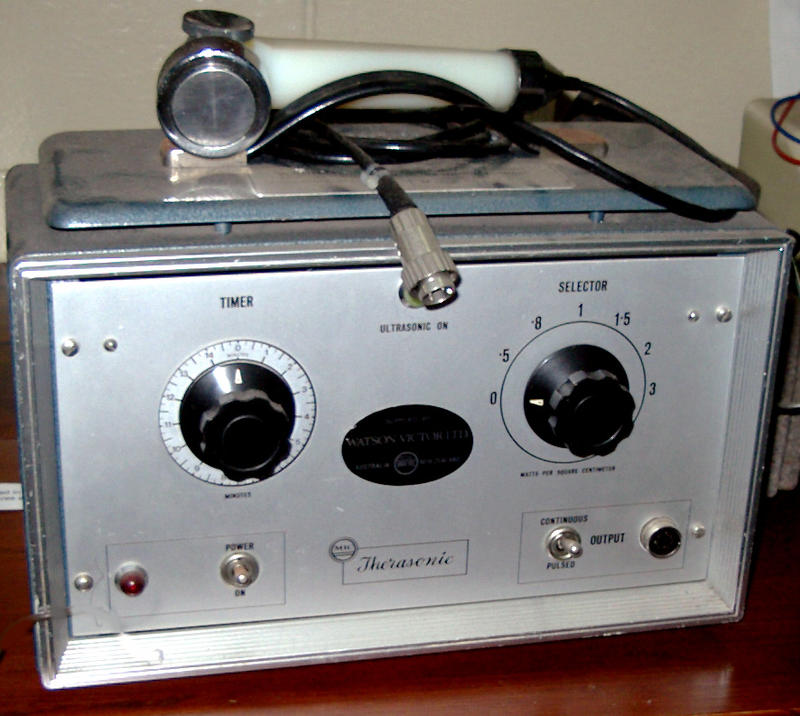The image is a detailed, color photograph of a vintage Therasonic Ultrasonic medical device, likely from the late 1950s to early 1960s. This silver piece of equipment, showing signs of wear and some chipping paint, is set on a dark wooden table. The front face of the machine features several controls: a dial in the upper left corner, a timer knob in the center-left, and a selector dial in the upper right, possibly to control output. Below these, there is a power switch and another operational switch. A distinctive element of the machine is the handheld sensor, resembling a white-handled sprinkler with a chrome nozzle, resting on top. This sensor is connected to the machine via a coiled black cord. The name "Therasonic" is visible at the bottom, with "Ultrasonic" noted at the top, indicating its purpose as an ultrasonic scanner, possibly used for medical diagnostics. Despite its dusty appearance and scuff marks, the device appears to be in generally good condition.